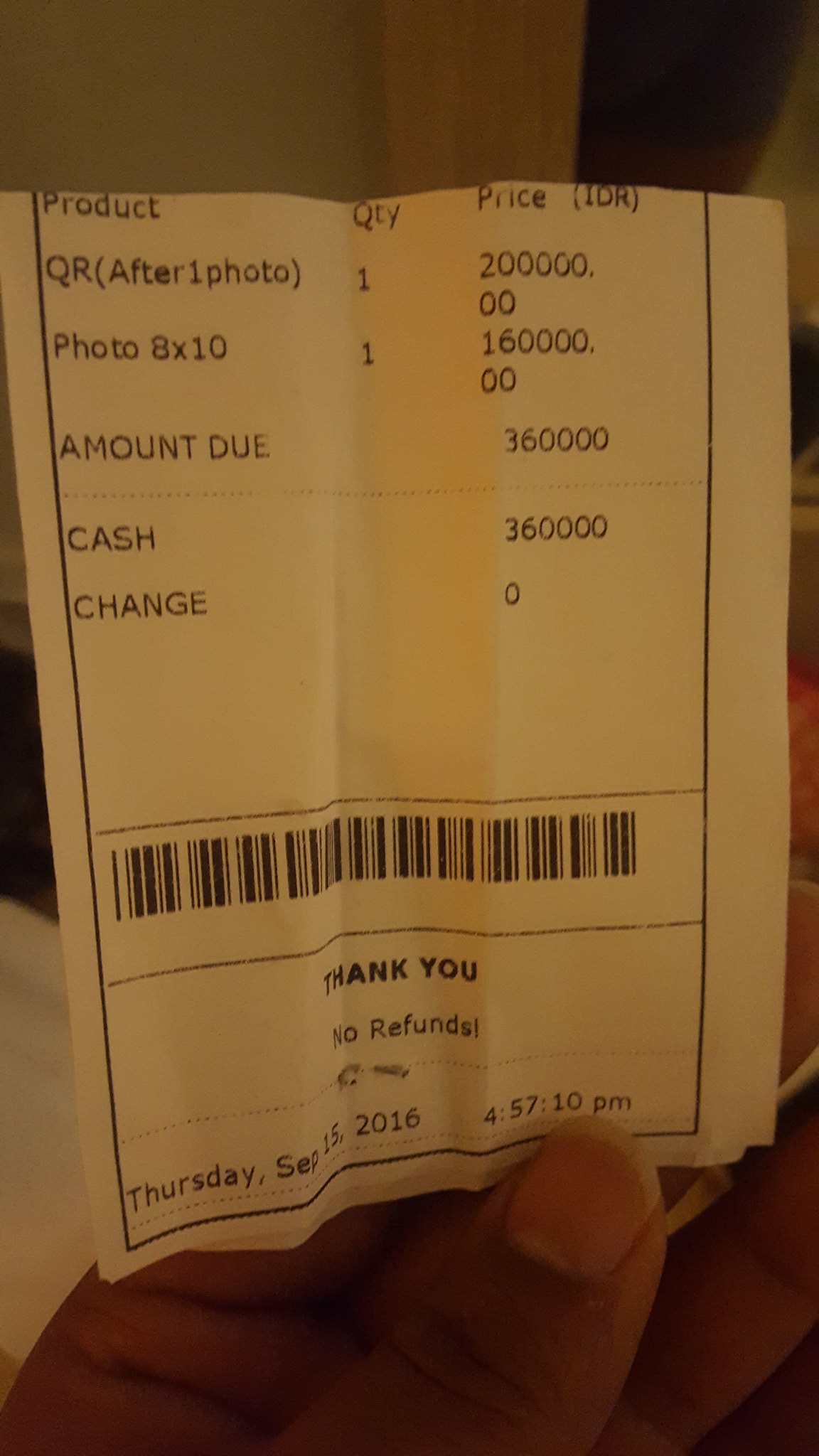In this vertical photograph, a hand is prominently featured at the bottom, clutching a crumpled receipt. The image offers a clear view of the person's thumb, including the nail, and the underside of their fingers as they carefully hold the paper. The text on the receipt details a transaction, listing "Product Quantity Price (IDR)" followed by the items purchased. Specifically, it mentions a QR code with a quantity of one, priced at 200,000.00 IDR, and an 8x10 photo costing 160,000.00 IDR. The total amount due is noted as 36,000.00 IDR, indicating a payment made in cash without any change. A barcode and a "Thank You" note, specifying "No refunds," are printed at the bottom. Additionally, the date and time of the transaction are stamped as Thursday, September 15th, 2016, at 4:57:10 p.m. While the receipt uses the abbreviation IDR, the currency is unspecified within the context of this caption.